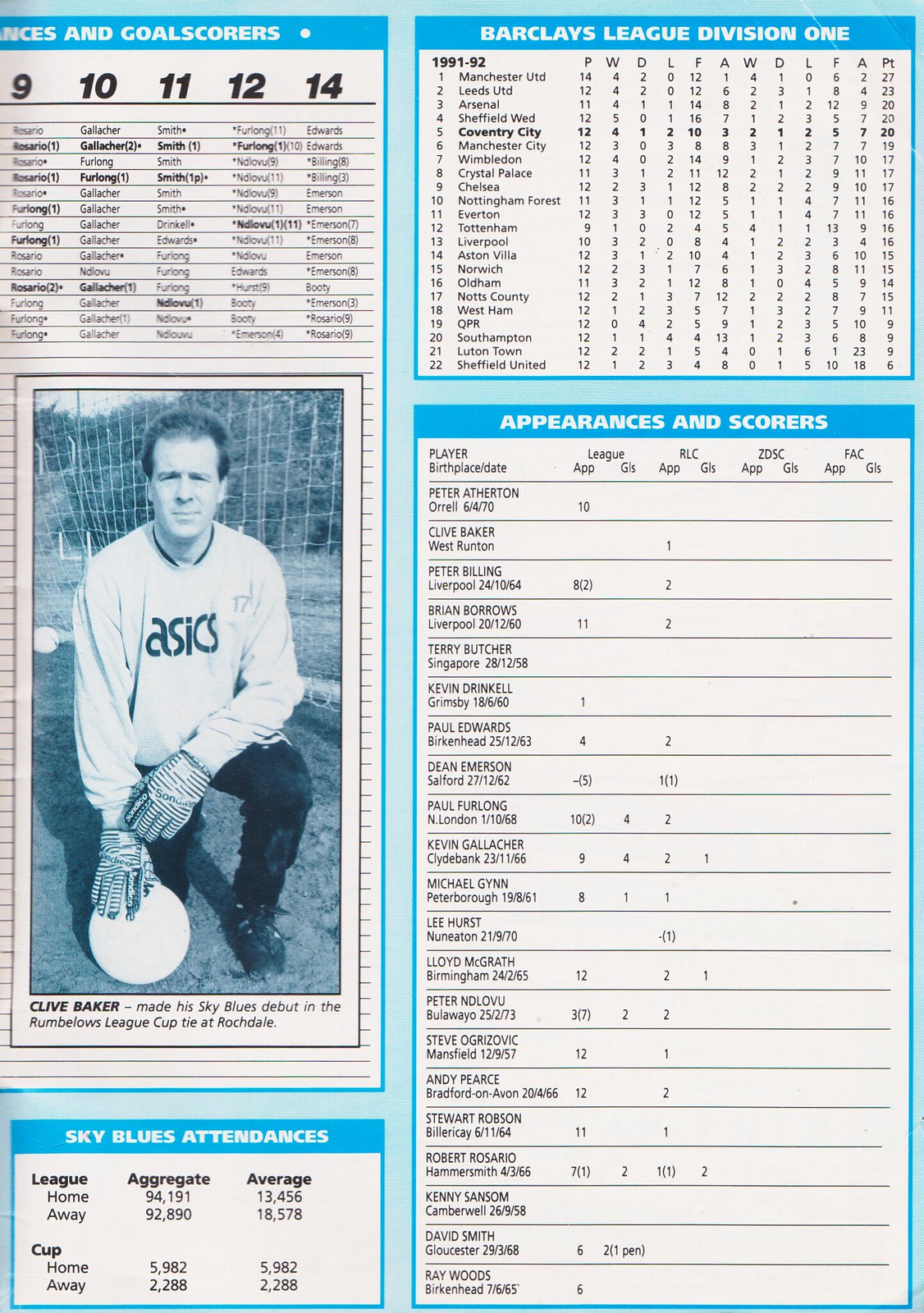The image is a rectangular snippet, likely from a magazine or the back of a playing card, focusing on a soccer team's statistics. Dominating the left upper corner are bold numbers 9, 10, 11, and 12 set in black against a white backdrop. Beneath this section, there is a black and white photograph of Clive Baker, a footballer, kneeling on the ground with a ball in his right hand and the net behind him. He is identified as a goalie, wearing a white long-sleeved jersey with gloves and black pants.

To the right of the photograph, detailed statistics and information about the Barclays League Division 1 season from 1991 to 1992 are prominently displayed. This includes team names like Manchester United and Leeds United, along with their scores, league standings, and player scoring statistics printed in small black text. Another highlighted section is titled "Appearances and Scorers," listing players' names and their performance stats.

Finally, towards the bottom right, a box labeled "Sky Blues Attendances" provides detailed aggregation of attendance figures for league and cup matches, presented in blue text on a white background. The overall layout is dense with information, blending scores, player stats, and attendance figures, particularly appealing to enthusiasts familiar with soccer terminology and history.